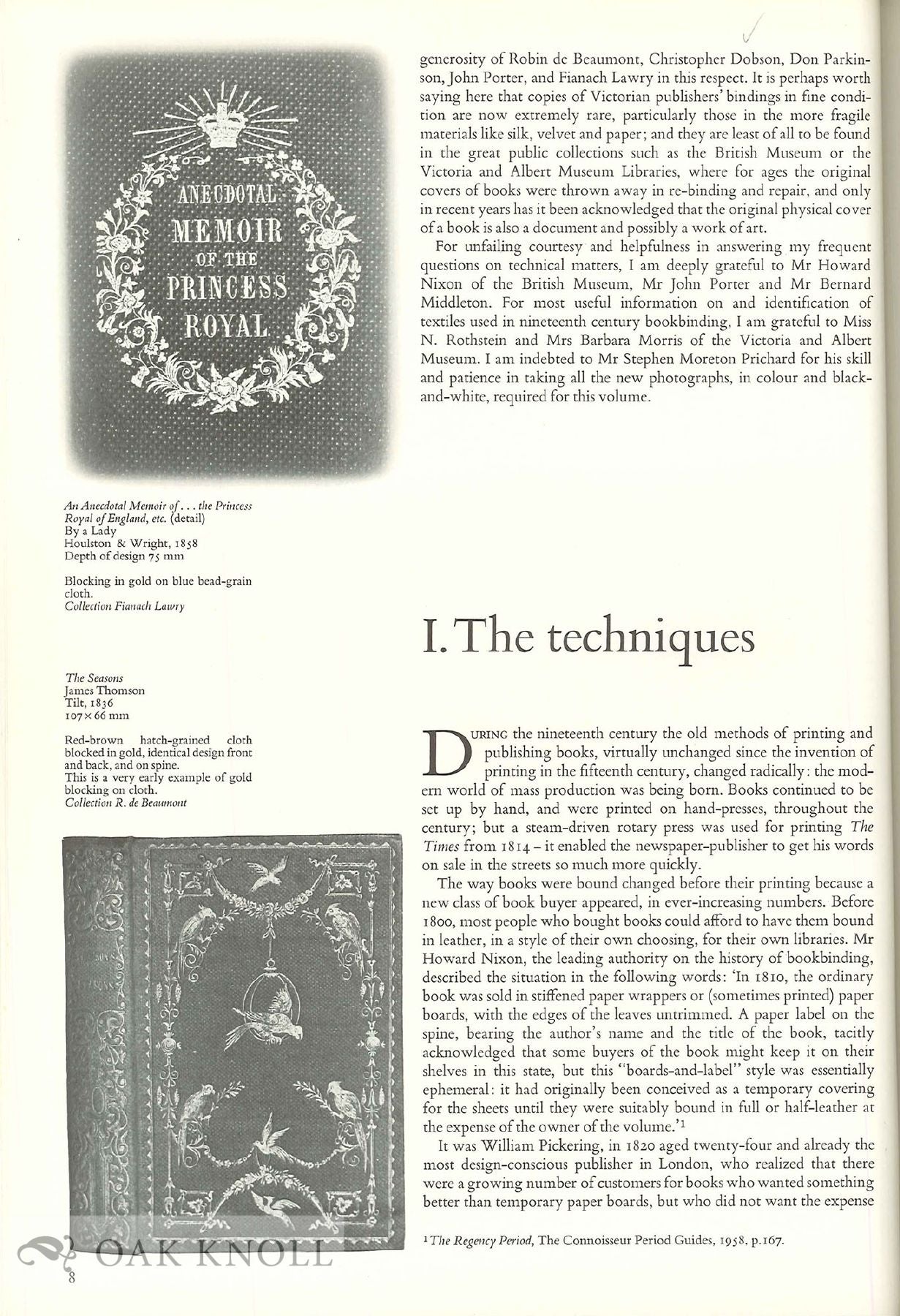The image is a scan of an off-white, almost yellowish page from an old book or magazine, divided into two sections. On the left side, there are two black and white pictures: the upper picture features a circular design with text inside that reads "Anecdotal Memoir of the Princess Royal," and the lower picture shows a rectangular design. Between these images, there is some explanatory text. The right side of the page contains a considerable amount of text organized into four or five paragraphs. This text discusses the evolution of printing and bookbinding in the 19th century, mentioning how the introduction of steam-driven rotary presses in 1814 revolutionized the speed at which newspapers, specifically The Times, were published. The text also highlights changes in bookbinding practices due to the emergence of a new class of book buyers who could not afford custom leather bindings for their libraries. The leading authority on bookmaking history, Mr. Howard Nixon, is quoted. Additionally, there is a watermark in the bottom left corner that reads "Oak Knoll."